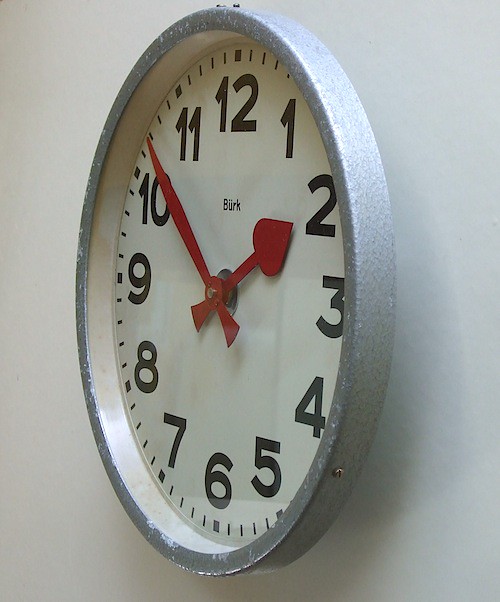The image depicts a round wall clock with a silver aluminum frame, slightly tilted diagonally on a white wall. The clock features a white face with black numbers ranging from 1 to 12, clearly marking the hours. Centered below the 12 o'clock position is the brand name "Burke" in black lettering. The clock is equipped with two red hands: the hour hand resembling a spade and the minute hand resembling a sword. Both hands indicate the time as 1:52, with the hour hand pointing towards the 2 and the minute hand two notches past the 10. The clock's simplistic design is further accentuated by a clear plastic cover, providing an unobstructed view of its face. The image is captured from a slight side angle, making the "3" on the clock appear closer to the viewer than the "9."